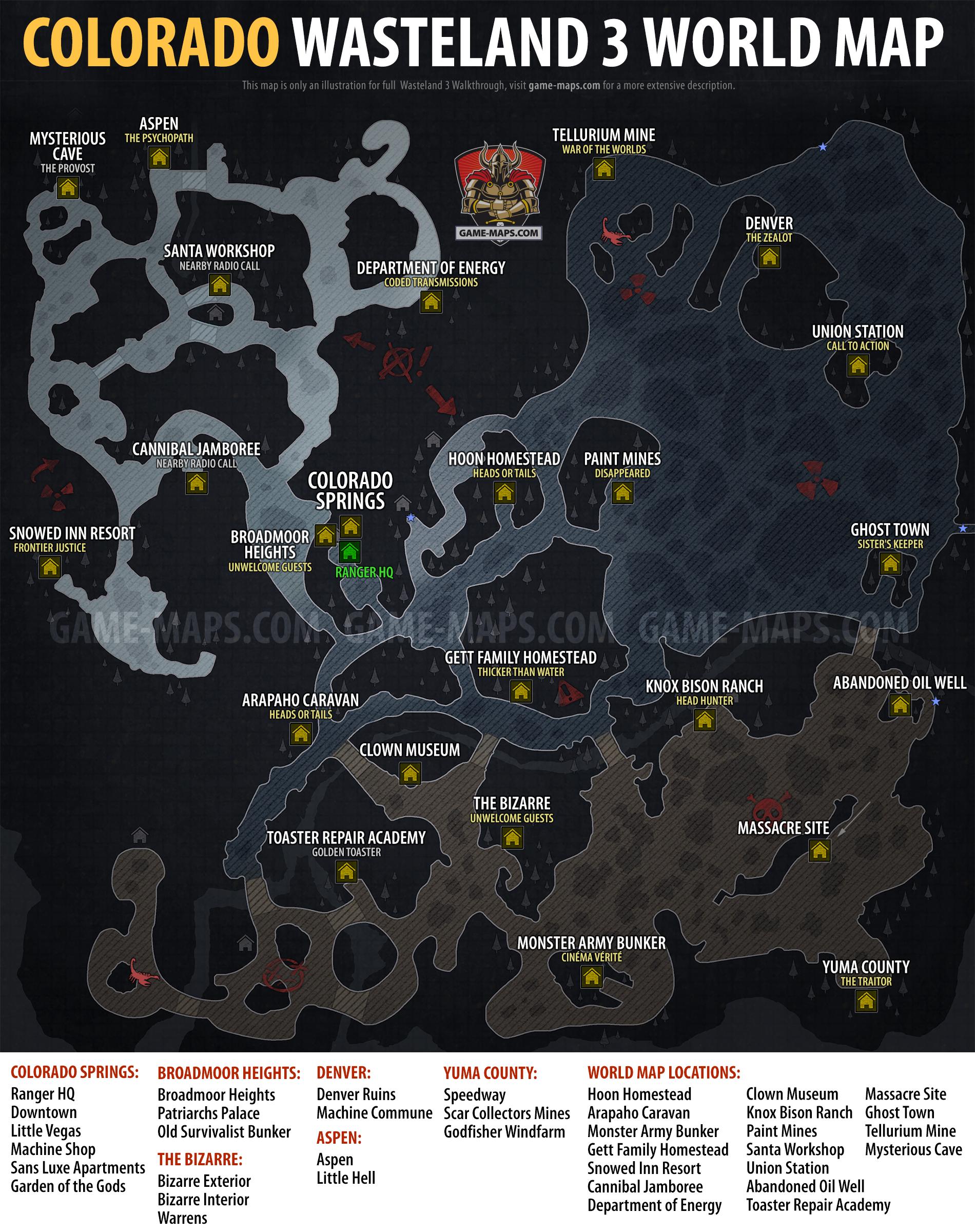The image is a detailed, overhead map entitled "Colorado Wasteland 3 World Map," indicating it's likely from a game set in a post-apocalyptic version of Colorado. The map features a mix of real and fictional points of interest, creating a rich and varied landscape. Notable locations include Denver, Union Station, and Colorado Springs, alongside more imaginative sites such as Santa's Workshop, Cannibal Jamboree, and the Toaster Repair Academy. Additional places marked on the map are the Department of Energy, Moon Homestead, the Bazaar, Clown Museum, Ranger Headquarters, and an Abandoned Oil Well. The map also includes mysteriously labeled areas like the Yuma County Massacre Site and Broadmoor Heights. Surrounding these locations are possibly significant, yet unclear, symbols and swirls, along with an oversized depiction of a lake, adding to the map's post-apocalyptic aesthetic and mystique.